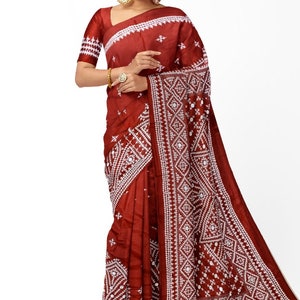The image depicts a cropped photograph of a woman, whose head is out of frame, modeling a traditional Indian dress. She is adorned in a dark sunset red sari with intricate white thread designs. The background gradients from solid white on the left to a cream color on the right. The sari features ornate white patterns across the chest, a bold white ribbon or stripe design, and further embellishments on the arm bands and under the chest ribbon. The right sleeve of the sari reaches down to her elbow, while the left side is draped elegantly over her arm, showcasing an elaborate white decorative pattern. She accessorizes with a circular ring on her left index finger and a bracelet on her right wrist.